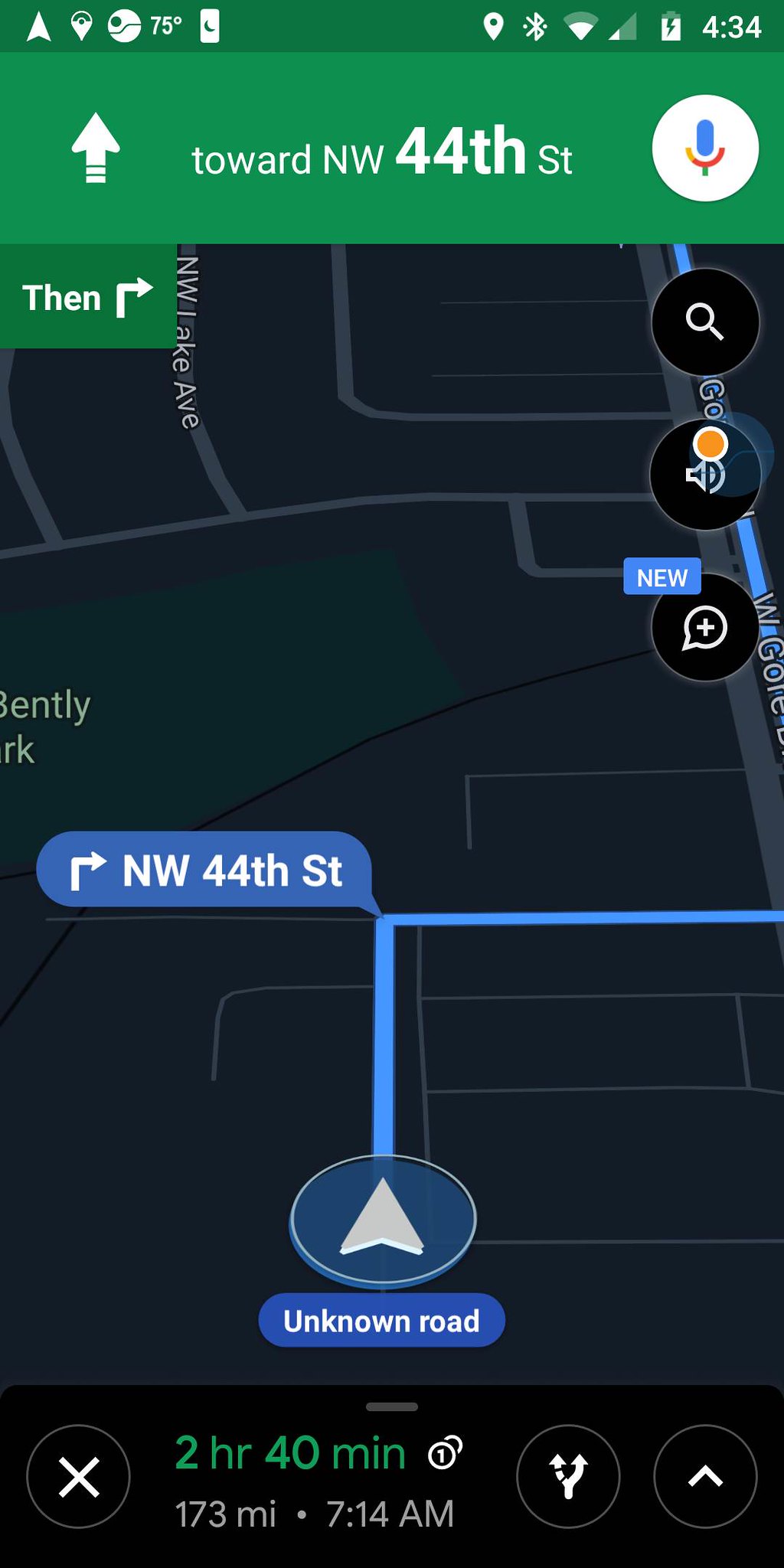This detailed image of Google Maps occupies the entire frame without any borders. The map display features a palette of black, blue, green, and white. At the top of the image, the text reads "Toward Northwest 44th Street" in green, black, and white fonts. On the right side of the screen, there are four distinct icons: a microphone for voice commands, a zoom-in feature, an audio icon, and a "New" icon featuring a plus sign. On the far left, an upward-pointing arrow accompanies the text "Toward Northwest 44th Street." 

In the middle of the image, a turning signal icon indicates a right turn, paired with the text "Northwest 44th Street" displayed in blue and white. Additionally, beneath the directional information, a blue banner with white text conveys travel details: "Towards Unknown Road, 2 hours 40 minutes, 173 miles, 7:14 a.m." The image combines various map and navigation details, giving a comprehensive view of the route and related information.